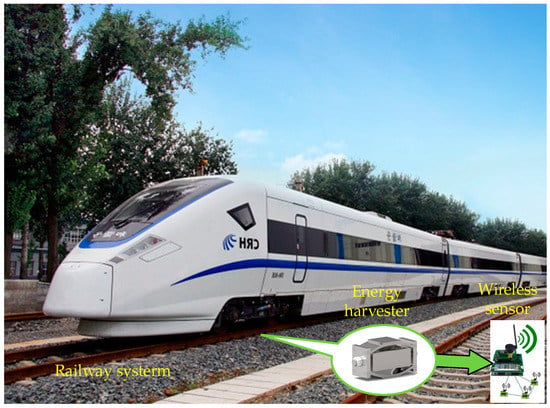In this vividly captured photograph, we see a sleek, modern train moving from the right towards the left, with its nose almost reaching the left edge of the frame. The train, predominantly white, boasts a striking royal blue stripe that runs horizontally just beneath its windows, adding a touch of elegance to its streamlined appearance. The shot is set outdoors on a sunny day, with a brilliant blue sky adorned by a few light, wispy clouds. In the background, lush green trees are bathed in sunlight, enhancing the scenic beauty of the scene.

At the bottom of the photograph, yellow text labels provide additional information. To the left, it reads "Railway Sisterm," likely a typo for "Railway System." Another label states "Energy Harvester and Wireless Sensor," suggesting an innovative technology aspect related to the train. Additionally, there is an illustrative diagram resembling a white speech bubble outlined in green, featuring a gray device inside it, potentially depicting the aforementioned energy harvester and wireless sensor. This detailed and informative caption brings clarity and context to the image, highlighting the train's modern design and the technological advancements associated with it.